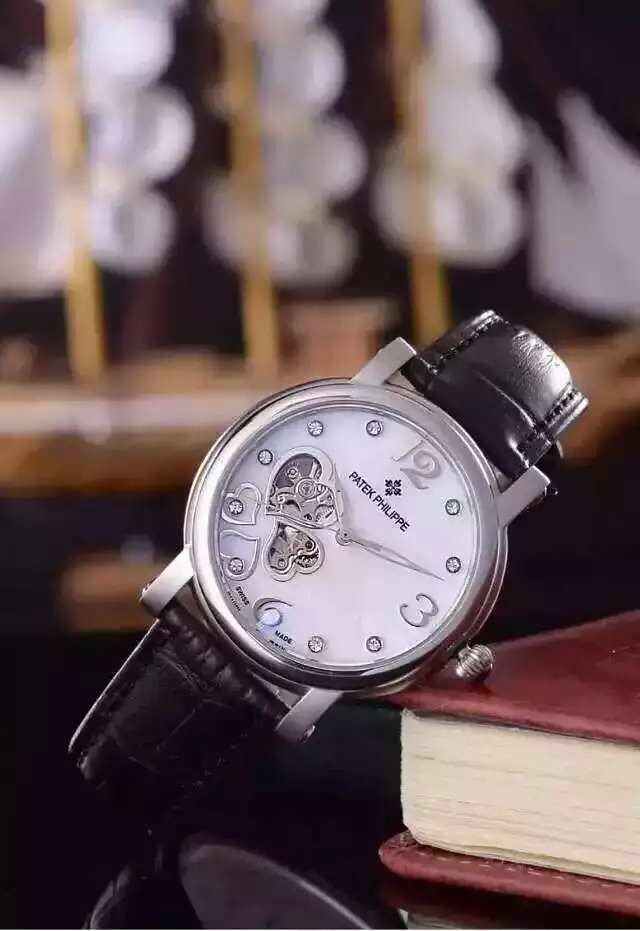This color photograph, captured in portrait mode, showcases a luxurious Patek Philippe watch with meticulous detailing. The watch, featuring a white face, is positioned diagonally across a book, leaning from the upper left to the upper right corner. Its platinum dial is adorned with platinum numerals at 12, 3, and 6, while the remaining positions are marked by sparkling diamonds. Notably, the left side of the watch displays four heart-shaped platinum elements, with two hearts offering a glimpse into the inner workings, reminiscent of delicate time-keeping clovers. The watch, complete with a dark leather strap embellished with black stitching, bears the name "Patek Philippe" inscribed from the top to the bottom right. Below the 6, the dial reads "Swiss made." The watch rests on a brown leather-bound book with white pages, which lies on a black table. The background is artistically blurred, with hints of white, fluffy floral elements on light brown stems, adding an elegant depth to the scene.